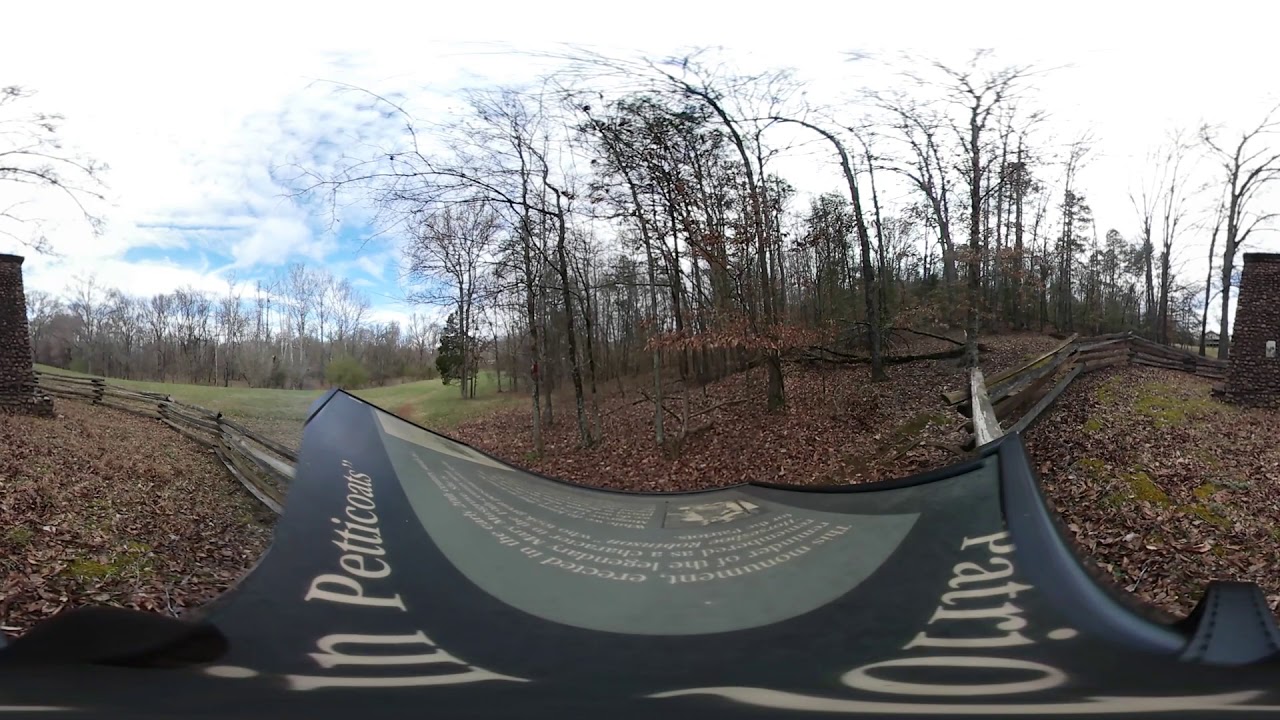The photograph captures a distorted, panoramic view of a largely barren forest scene taken during the fall or winter. The image shows a forest with numerous trees that have lost most of their leaves, indicated by the thick layer of brown leaves scattered across the ground. A mix of evergreen trees is visible in the background, providing a hint of green amidst the predominantly bare branches. The sky above is mostly cloudy, with patches of light blue peeking through, suggesting a partly to mostly cloudy day. Prominent in the image are wooden split rail fences stretching to either side, framing the scene. A small brick or stone building, described as a stone house or tower, is situated nearby, accompanied by an open grass field in the background. In the center of the photograph, a blue sign with white letters stands out, reading "IN Petcoats." The overall view is slightly skewed and squashed, contributing to the panoramic distortion of the image.